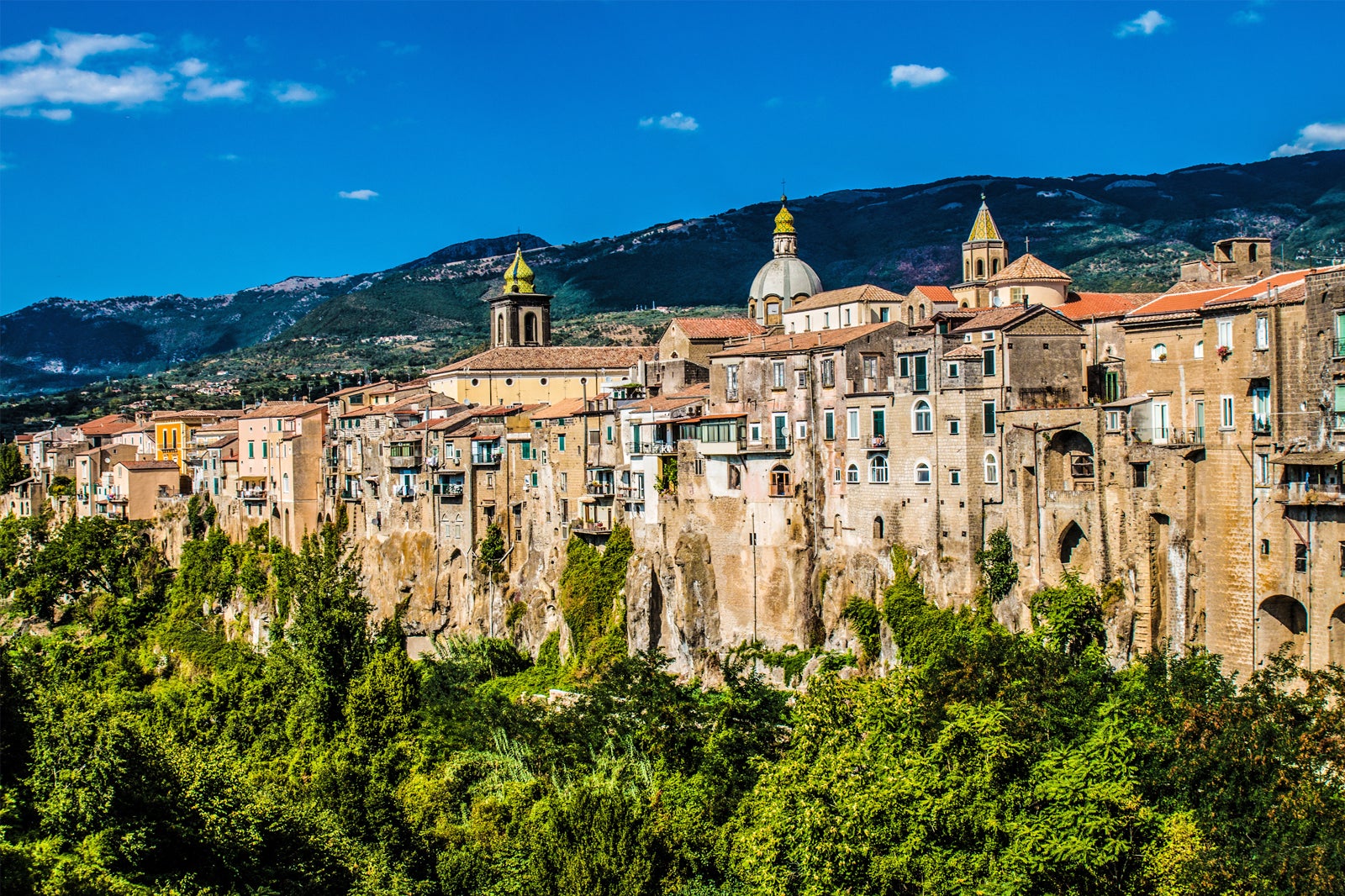This modern-day photograph captures an ancient, European-style city nestled within a mountainous landscape. The city, characterized by its impressive stone walls, appears to be integrated into the very fabric of these fortifications. Dominated by tan and brown hues with white window borders, the buildings exhibit centuries-old architectural features, including tall, aged structures with numerous archways. Prominently, three distinct steeples punctuate the skyline: a rounded one at the center, a missile-shaped one to the right, and another similarly missile-shaped on the left. These steeples, likely belonging to churches or cathedrals, rise above the cityscape, glistening with golden accents. In the foreground, a verdant forest stretches upwards, offering a contrast to the urban spread. The crisp, clear sky overhead is painted a light blue, interspersed with small, white clouds, framing this timeless scene against a backdrop of distant, rugged mountains.